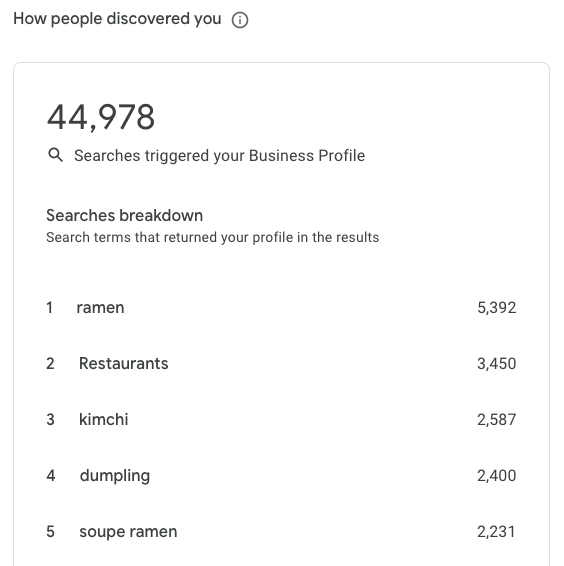This detailed caption provides a clear breakdown of how search terms contribute to the visibility of a business profile, accompanied by a visual aid involving specific search terms and their related metrics.

---

"An analytic chart showcasing how users discovered the business profile via various search terms. At the center, a magnifying glass icon highlights 'Searches Triggering Your Business Profile,' with a total of '44,978' searches. The detailed breakdown includes the following search terms: 'Ramen' with 5,392 searches, 'Restaurants' with 3,450 searches, 'Kimchi' with 2,587 searches, 'Dumplings' with 2,400 searches, and 'Super Ramen' with 2,023 searches. The image has a clean white background, emphasizing the text and metrics, and visually representing the importance of these search terms in driving visibility and engagement."

---

This in-depth caption not only explains the image but also contextualizes the data, making it easier for the viewer to comprehend the significance of each search term.